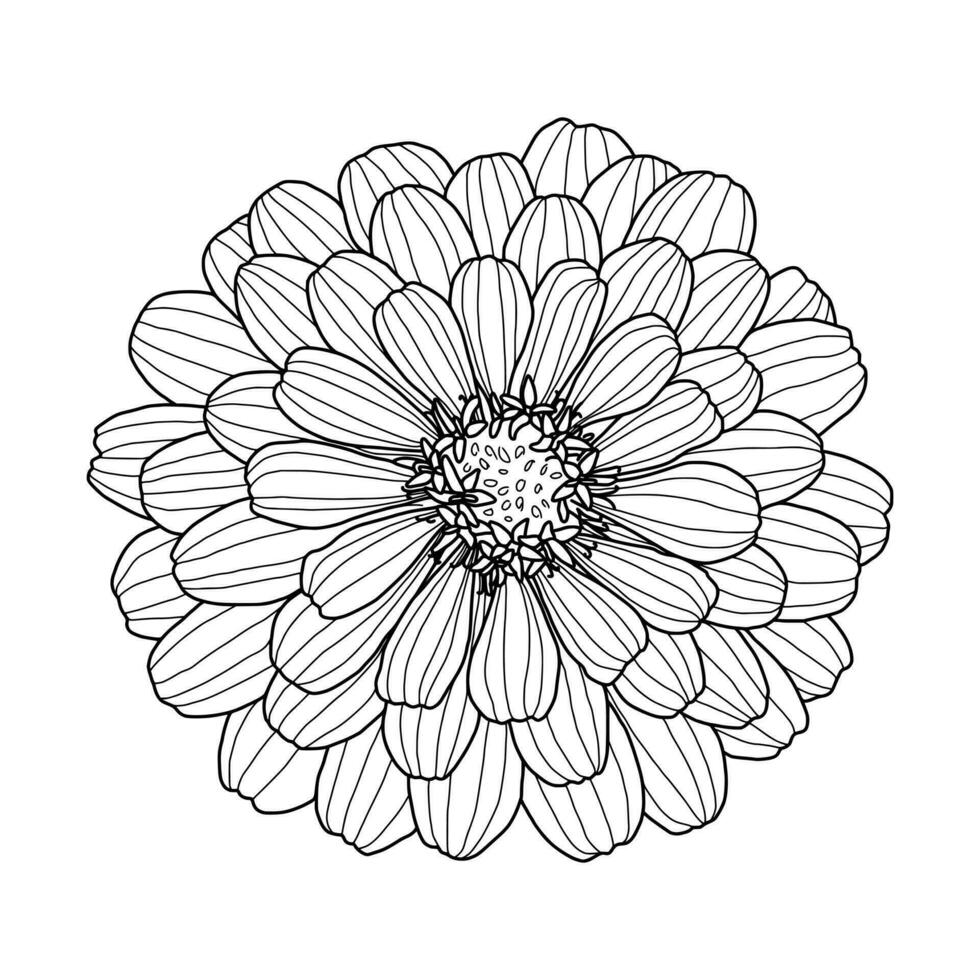This is a highly detailed black and white outline drawing of a dahlia flower, rendered with precision and clarity. The image, which resembles a page from a coloring book, is set against a pure white background, emphasizing its monochromatic nature. The flower features four concentric layers of petals, each meticulously outlined in black. The petals grow progressively longer from the innermost layer to the outermost layer. Each petal is intricately detailed with four lines extending from the flower's center to the tips of the petals. At the heart of the dahlia, small lines and dots depict the central pistil and pollen, adding to the drawing's realism. The topmost layer of petals showcases approximately thirteen petals, with the subsequent layers expanding outward in size and number. No stem is featured, keeping the focus entirely on the top-down view of the flower. The repetitive patterns and lack of color suggest this artwork is intended for coloring, inviting the viewer to bring the flower to life with their own palette.